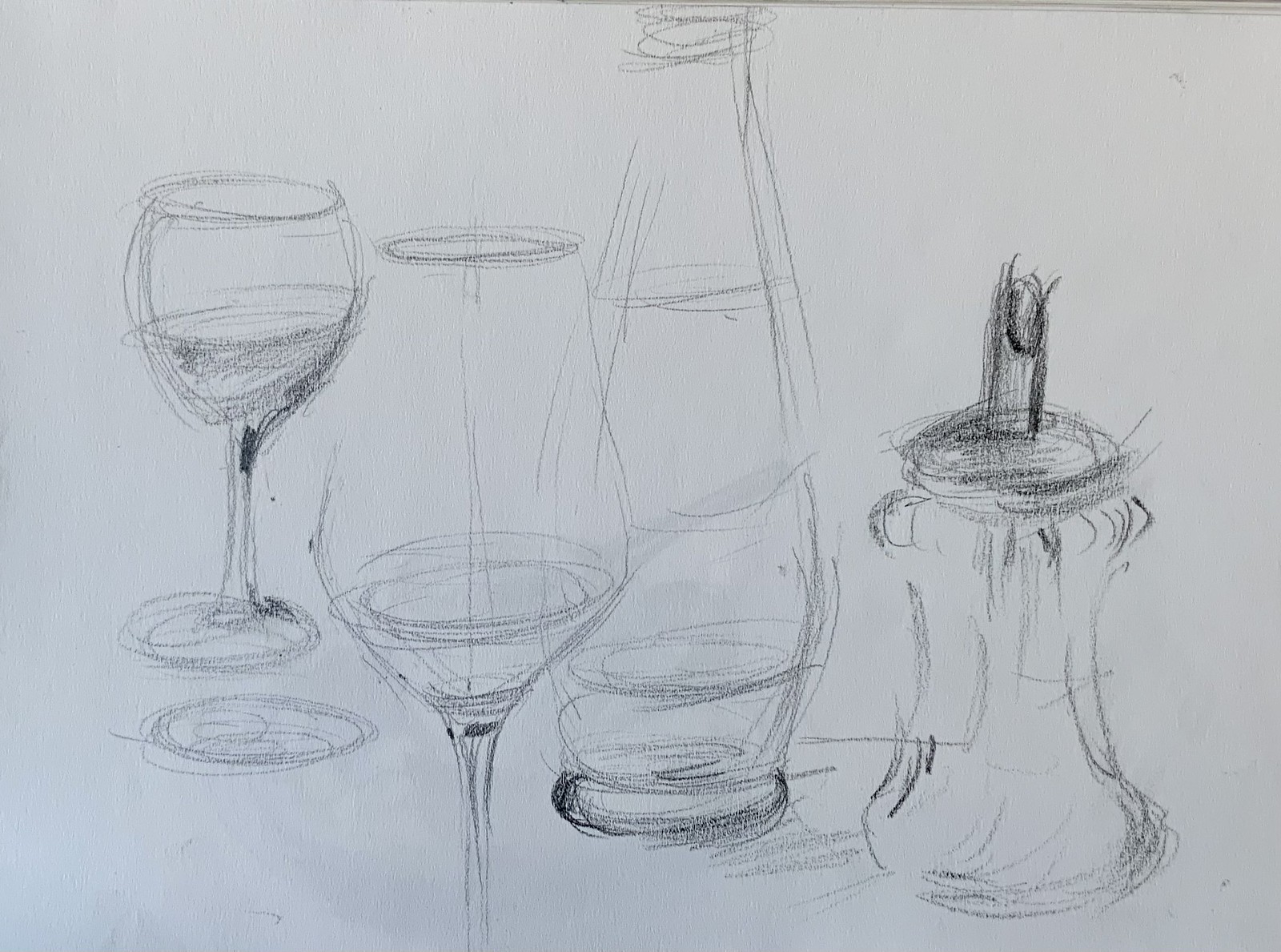The image is a meticulously drawn, black-and-white sketch on a rectangular piece of paper, oriented horizontally. The background consists entirely of the white paper, with the drawing executed in charcoal or pencil marker. The scene depicts a still life setup of various glassware and containers, possibly observed on a table in a restaurant or home. 

On the far left, there's a half-filled, shorter-stemmed, rounded wine glass. Moving toward the center, a taller, fluted wine glass is depicted, containing a smaller amount of liquid. Behind these glasses, a large, empty carafe or bottle, possibly a water bottle, stands prominently. 

On the far right, there's a cylindrical object with a metallic pour spout affixed on top; this could be a sugar dispenser with a screw-top lid designed for dispensing precise amounts, similar in measurement to a teaspoon. 

The sketch is detailed, emphasizing the textures and forms of the items through careful shading and line work, capturing a quiet, contemplative moment with elegant simplicity.